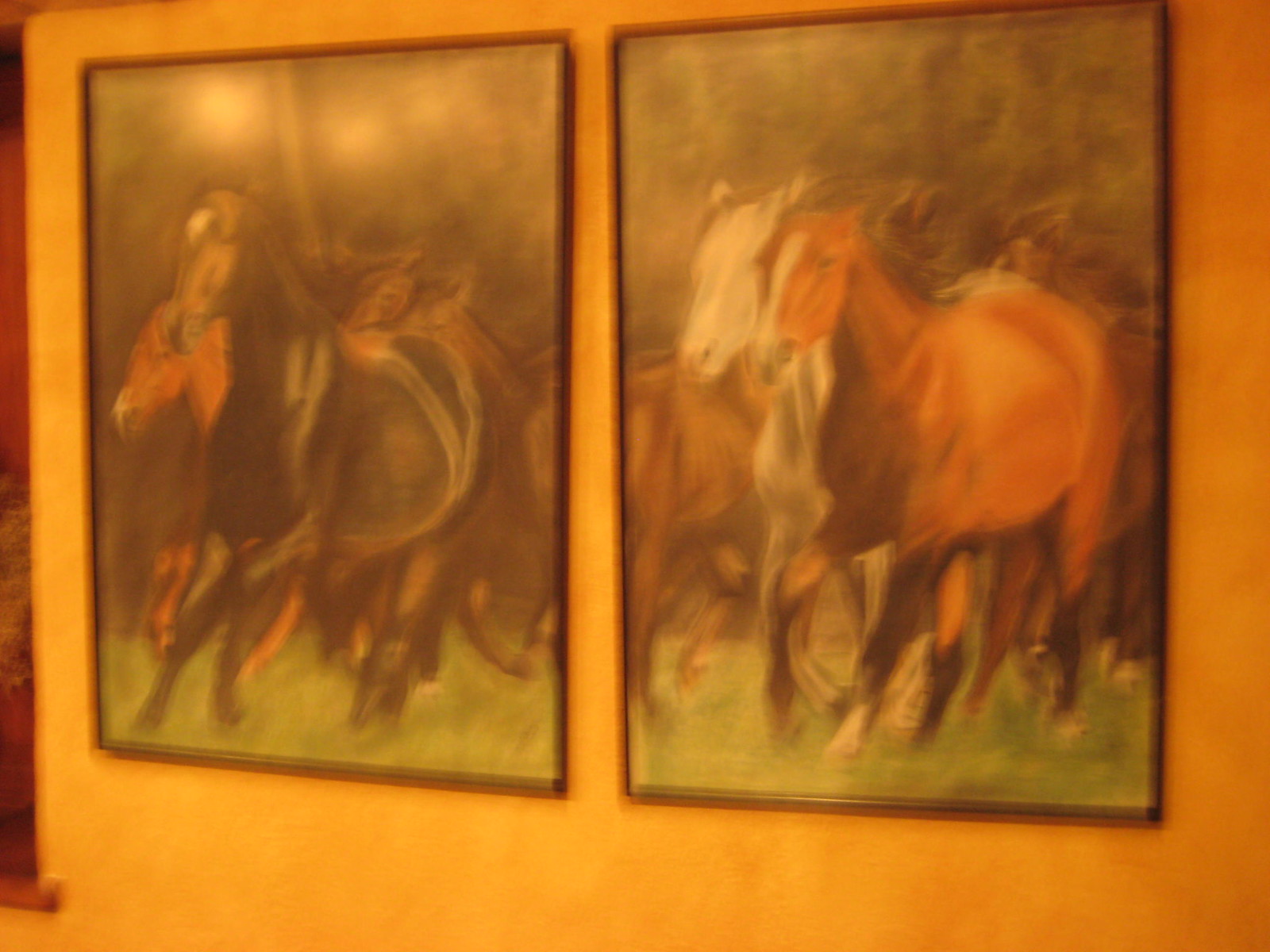This is a photograph of two portrait-style paintings hung side-by-side on a yellow or light orange wall, although the wall color might be distorted due to the photograph's poor quality. The photograph is blurry and out of focus, making it difficult to discern fine details. The paintings, each framed with a thin, dark border, depict a natural scene with horses running freely on a green field against a blurred tree background. The left painting shows a black horse, a chestnut horse, and a dark brown horse with a white streak on its nose. The right painting features brown horses, including one with white markings and another with a white face. Together, these paintings resemble a single continuous scene, albeit separated by a small gap of about five centimeters. The loose, wispy brush strokes evoke a sense of movement within the paintings. Additionally, a scroll-like piece of art with a wooden hanger at the bottom partially obscures the far left of the wall. The paintings appear slightly misaligned, with the top edges closer together than the bottom ones.